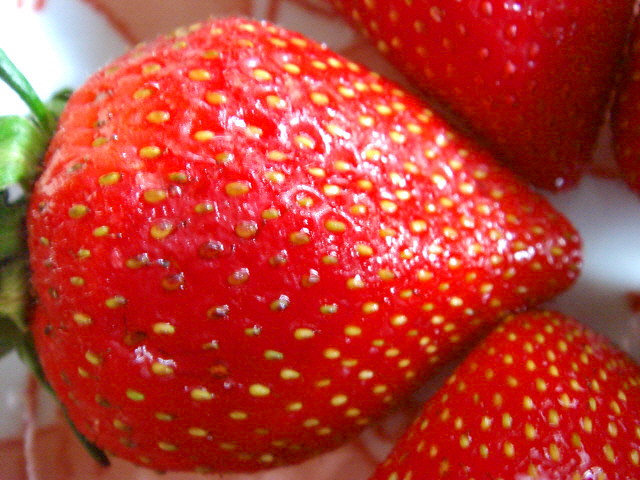This is an extremely detailed close-up photo of a bright, ripe strawberry, showcasing almost the entire fruit except for a small portion of the green stem at the top. The strawberry is laying on a white surface, with the creamy white background softly blurred to highlight the fruit's vibrant color. The main strawberry is a radiant strawberry red, glistening with juicy ripeness and studded with prominent yellowish seeds, some of which have a slight brownish-tan hue, giving it a natural and fresh appearance. Surrounding the main strawberry, there are parts of two other strawberries pointing towards its end; their seeds are a uniform yellow, adding to the delectable presentation. The strawberries' vivid red hues and the slight variations in their seeds' colors accentuate their perfect ripeness and delicious appeal, making the image mouthwatering. It beautifully captures the essence of fresh, ready-to-eat strawberries, making it irresistibly tempting.